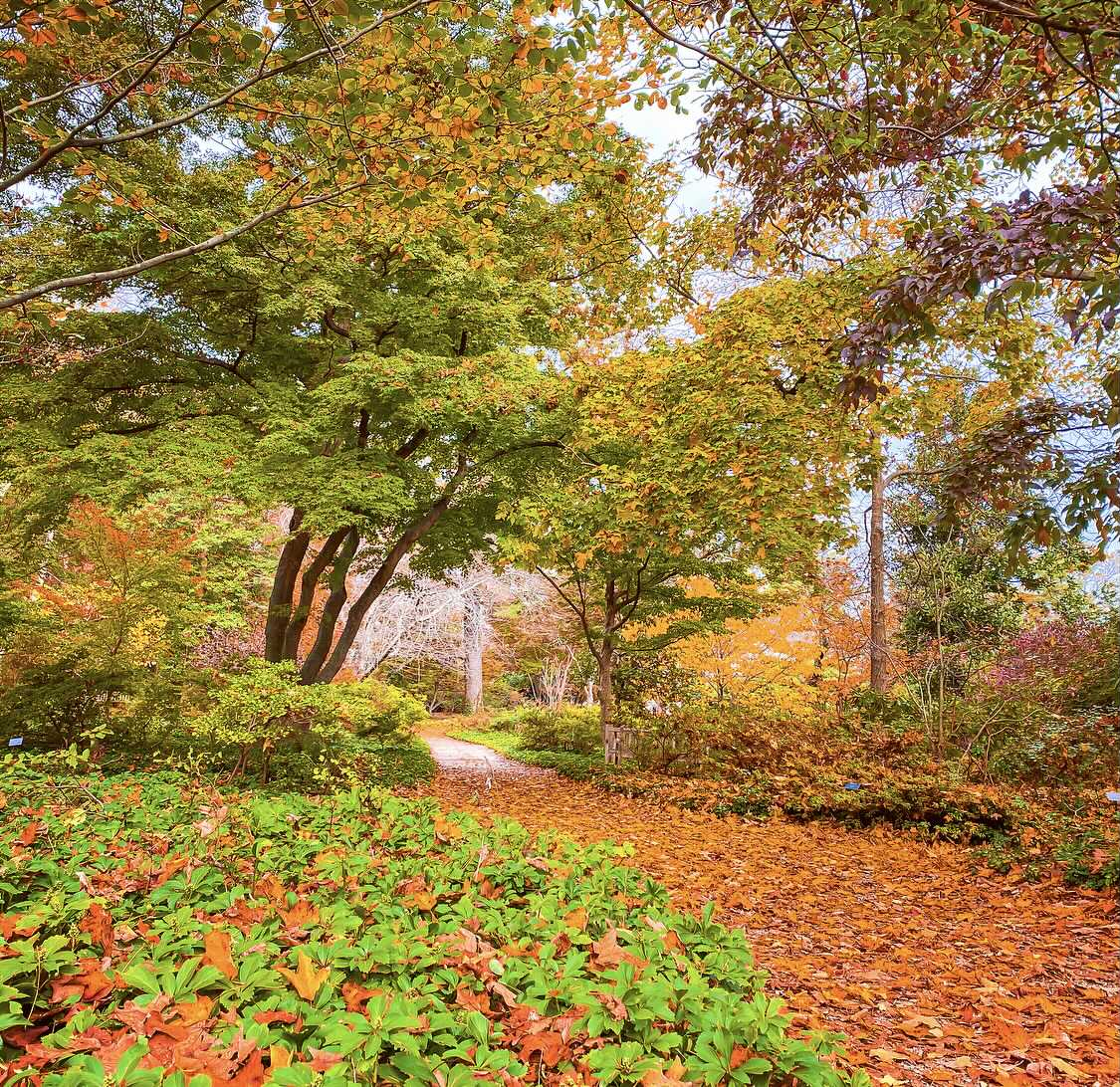This captivating autumn photograph showcases a lush forest blanketed with vibrant fall foliage. A well-trodden path runs through the center of the forest, almost obscured by a thick carpet of orange, red, and brown leaves. The canopy above is predominantly green, but many leaves are gradually adopting rich autumnal hues, ranging from bright oranges to deep reds and maroons. To the left stands a prominent tree with four large trunks, its leaves a light mossy green, while to the right, another tree displays darker, maroon foliage. The forest floor is dotted with patches of greenish weeds, adding to the diverse palette of colors. The intricate interplay of green, red, orange, yellow, brown, and even some purples in the top right corner suggests that the photograph was taken in a region that experiences distinct seasonal changes, potentially resembling the picturesque landscapes of the Northeast or Midwest. The scene evokes the beauty of a serene walking trail nestled in the heart of nature's fall splendor.